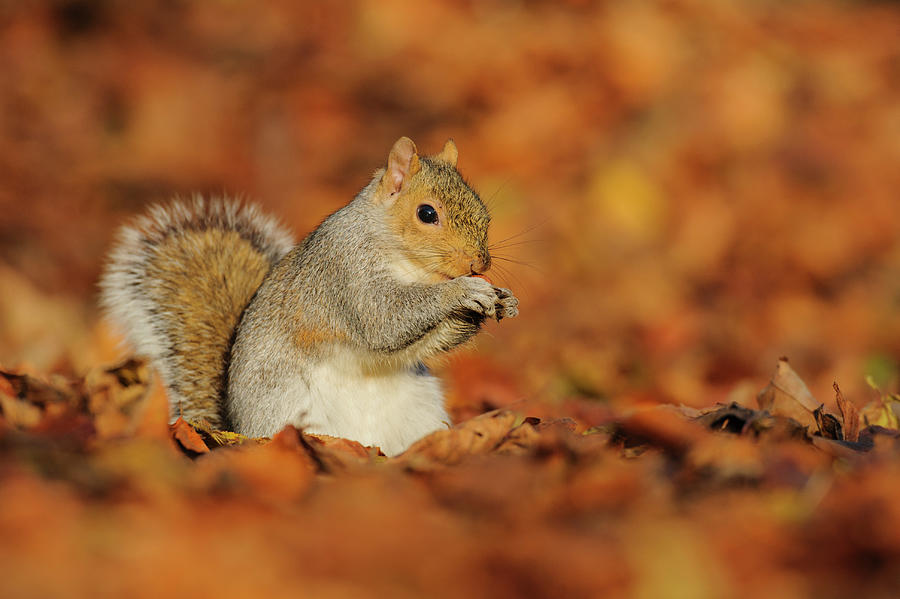This is a high-resolution color photograph taken outdoors during the day, capturing a charming moment of a gray squirrel amidst the autumn scenery. The squirrel, with a bushy tail and striking black eyes, sits upright on its back legs in a pile of crinkly fall leaves that display various shades of yellows, browns, reds, and oranges. Sunlight illuminates its beautiful white belly and gray back, while hints of reddish-tan fur add a warm touch to its face and tail, as well as being sprinkled throughout its coat. The squirrel is the main focus of the photograph, holding an acorn close to its mouth with its tiny raised paws, poised to take a bite. The background and most of the foreground are artistically blurred, drawing attention to the intricate details of the squirrel, including each individual whisker around its muzzle and above its eyes. This deliberate focus creates an intimate and endearing portrait of the squirrel in its natural, autumnal habitat.